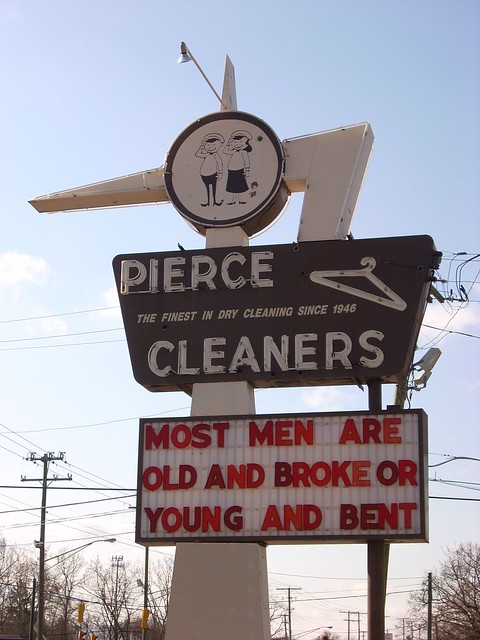This photograph captures a nostalgic advertisement for Pierce Cleaners, an old dry cleaning store likely originating from the 1950s or 1960s. The prominent sign is positioned along a city road and has a worn, aged appearance. At the top of the sign, there is a circular logo featuring a man and a woman dressed in sailor uniforms, possibly accompanied by a small child, rendered in a classic 1950s black-and-white cutesy art style. Below the logo, a broad, slightly asymmetrical sign bears the name "Pierce Cleaners" alongside the tagline, "The finest in dry cleaning since 1946," with an icon of a clothes hanger above it. At the bottom of the sign, in a rectangular box with replaceable letters, there is a humorous and perhaps hyperbolic message that reads, "MOST MEN ARE OLD AND BROKE OR YOUNG AND BENT." The backdrop features clear, cloud-free skies, with power lines, street lights, and leafless trees and bushes, situating the sign higher up and emphasizing its prominence in the landscape.